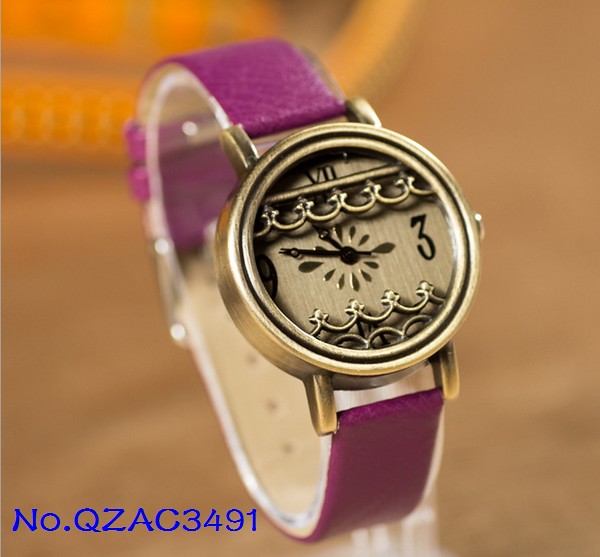A striking watch is showcased prominently in this photograph, with a softly blurred background that accentuates its detailed craftsmanship. The watch features a supple, purple band that could be made of leather or velvet, adding a luxurious touch. The circular face, encased in sleek silver steel, is elegantly adorned with black numerals. Roman numerals mark the 12 o'clock and 6 o'clock positions, while traditional numerals occupy the 9 o'clock and 3 o'clock positions. Two slender black hands glide over a sophisticated design of silver raindrop shapes within the watch face. The intricate detailing extends to engraved loops on the silver metal, gracefully overlaying the face and curving along the bottom, making the watch not only a timepiece but a work of art.